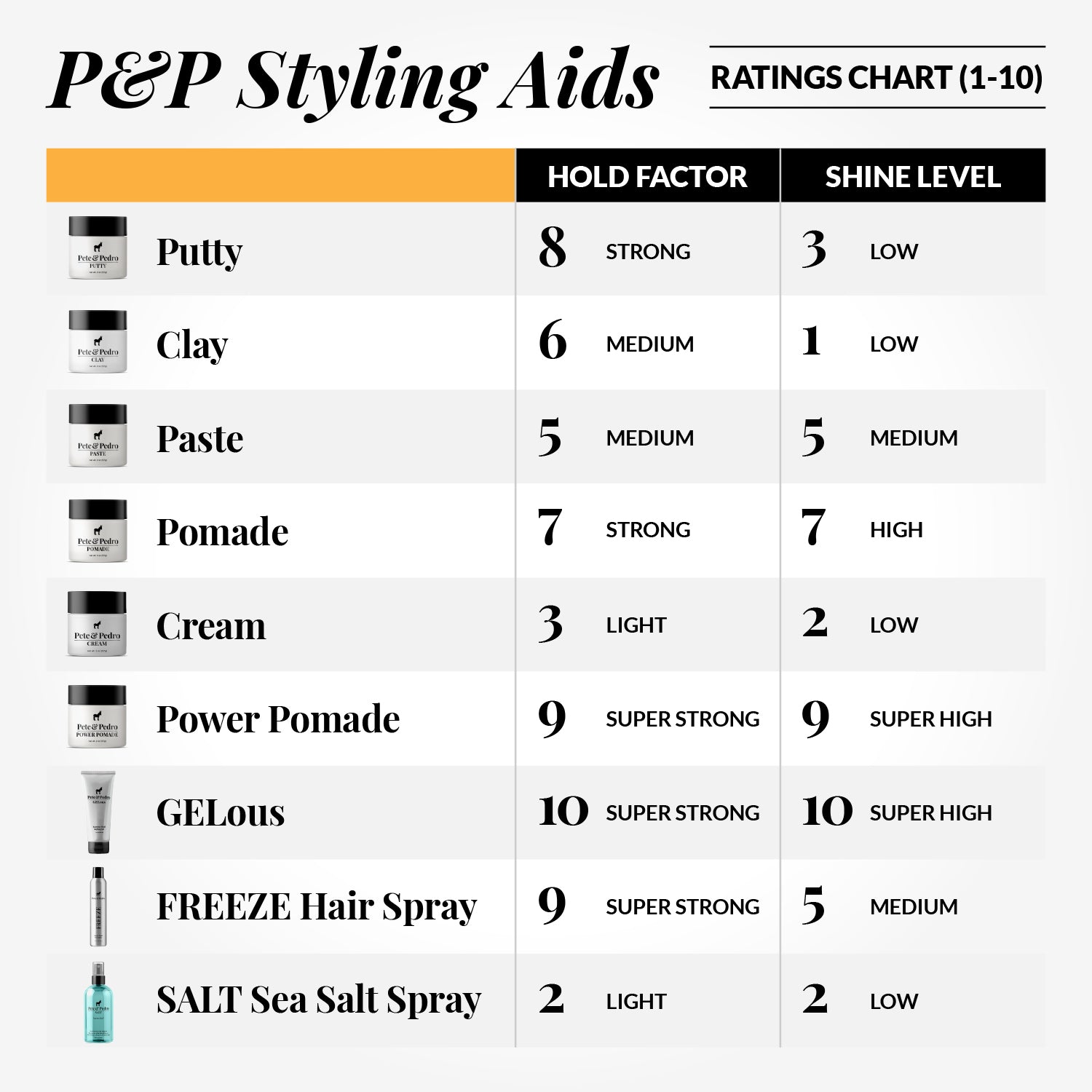This image is a detailed chart titled "P&P Styling Aids Rating Chart 1-10." Set against a white background, the chart is divided into vertical columns for different hair products, each rated by hold factor and shine level. The top section includes a black rectangle with the label "P&P Styling Aids" on the upper left and "Rating Trout 1-10" on the upper right. Just below this, a prominent yellow bar introduces the products listed as: Putty, Clay, Paste, Pomade, Cream, Power Pomade, Jealous (spelled G-E-Lous), Freeze Hairspray, and Sea Salt Hairspray. Each product's hold factor and shine level are indicated within black-bordered columns:

1. **Putty**: Hold Factor 8 (Strong), Shine Level 3 (Low)
2. **Clay**: Hold Factor 6 (Medium), Shine Level 1 (Low)
3. **Paste**: Hold Factor 5 (Medium), Shine Level 5 (Medium)
4. **Pomade**: Hold Factor 7 (Strong), Shine Level 7 (High)
5. **Cream**: Hold Factor 3 (Light), Shine Level 2 (Low)
6. **Power Pomade**: Hold Factor 9 (Super Strong), Shine Level 9 (Super High)
7. **Jealous**: Hold Factor 10 (Super Strong), Shine Level 10 (Super High)
8. **Freeze Hairspray**: Hold Factor 9 (Super Strong), Shine Level 5 (Medium)
9. **Sea Salt Hairspray**: Hold Factor 2 (Light), Shine Level 2 (Low)

"Jealous" is highlighted as the highest-rated product with the maximum scores for both hold and shine.